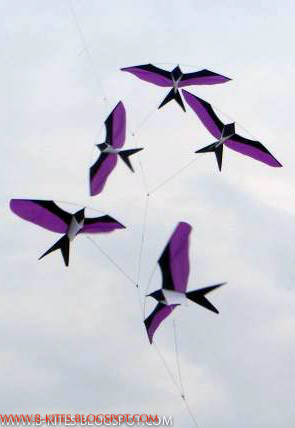The image is a detailed illustration of five bird-shaped kites soaring in the sky. Each kite is designed to resemble a swallow, with distinguishing features such as a black head, deeply forked black tail, and outstretched wings that fade from black at the forewing to purple on the edges. The bodies of the kites are predominantly white, and they appear to be flying against a very pale blue sky scattered with wisps of white clouds. The kites are interconnected by strings, creating the effect of a single, cohesive kite structure made up of these five swallow-shaped sections. Additionally, there are faintly visible wires that support the wings' shapes. At the bottom left of the image, watermarked in orange and white, are partially legible URLs, including "www.something-kitessomethingsomething.com" and "www.beekitesblogspot.com." The image also carries a watermark, making it clear that it is a curated illustration.